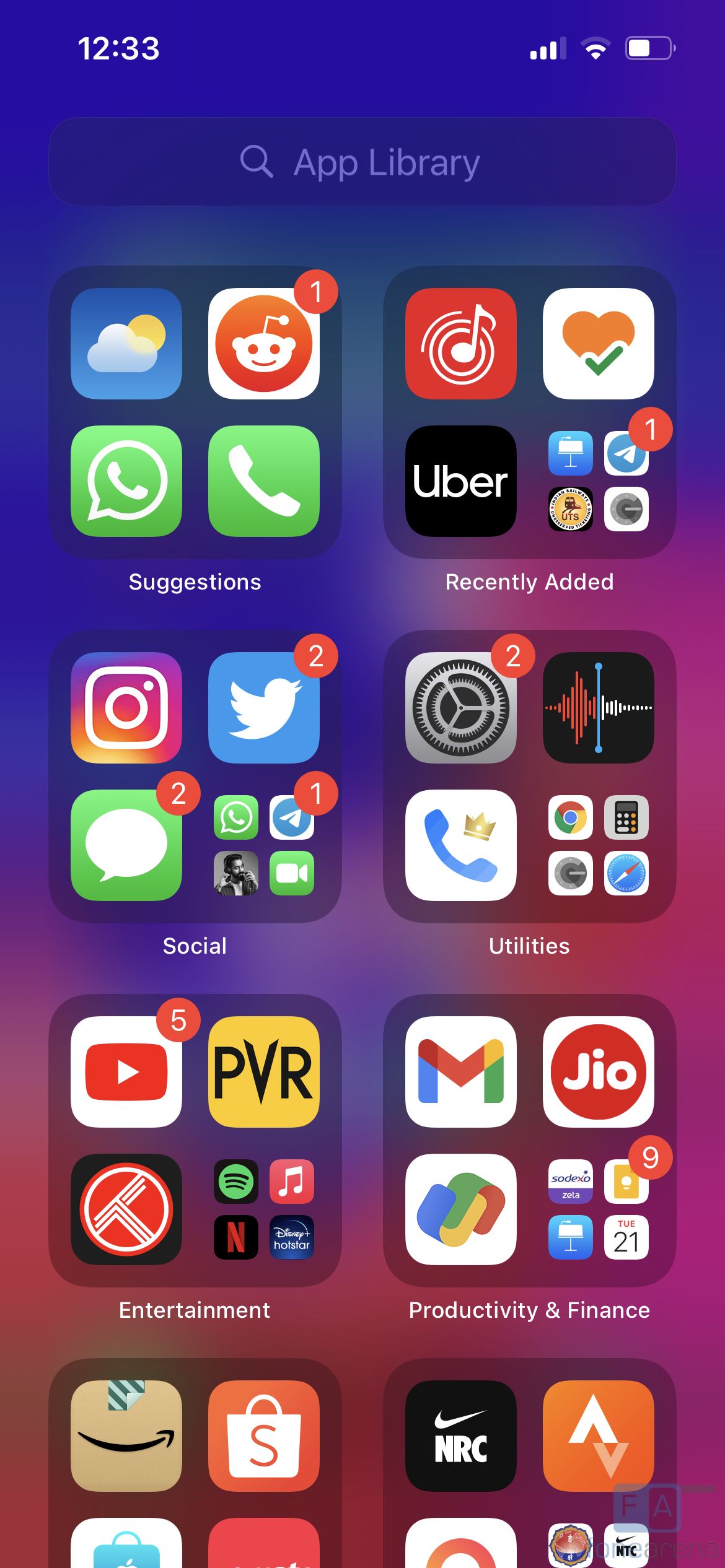A vibrant multi-gradient phone screen showcases a meticulously organized home page with various app folders. At the top, against a vivid purplish-blue background, the upper-left corner prominently displays "12:33" in white. The upper-right corner features three Wi-Fi bars, a Wi-Fi signal icon, and a battery icon indicating half battery life. Below, a white search bar labeled "App Library" with a search icon on the left stands out.

The home page is neatly arranged with eight folders, each containing four apps. The gradient transitions smoothly to pink towards the bottom of the screen. Each folder is labeled for easy navigation: "Suggestions" is on the top-left, with "Recently Added" on the top-right. The second row features "Social" on the left and "Utilities" to its right. The third row consists of "Entertainment" on the left and "Productivity & Finance" on the right. The labels of the two bottom-edge folders are off-screen and not visible.

Notably, several app icons within these folders have red notification bubbles, indicating between one to five pending notifications. This visually rich and highly organized layout exemplifies user efficiency and attention to detail.